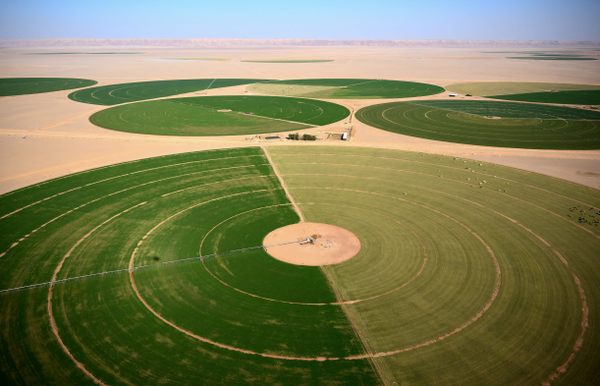In this captivating aerial photograph, we observe a striking landscape that seamlessly blends elements of a desert and fertile land. Dominating the foreground is a prominent circular pattern divided into two distinct halves: a darker lush green segment on the left, intersected by a brown line, transitioning into a lighter green on the right. Centrally located within this large circle is a smaller tan circle, seemingly the nucleus of this intriguing design. Surrounding this main feature, the landscape is dotted with numerous similar circular formations, each mirroring the split-tone and central circle arrangement. The circular areas are set against a backdrop that appears to be sandy or dirt-laden terrain, reminiscent of a desert. As the eye moves toward the horizon, the vast expanse reveals faint horizontal green lines that grow thicker and form more circular shapes, suggesting a highly organized agricultural pattern or possibly irrigation fields. The image's upper portion beautifully contrasts this structured greenery with a clear, light blue sky, enhancing the overall sense of vastness and symmetry in this mesmerizing scene.